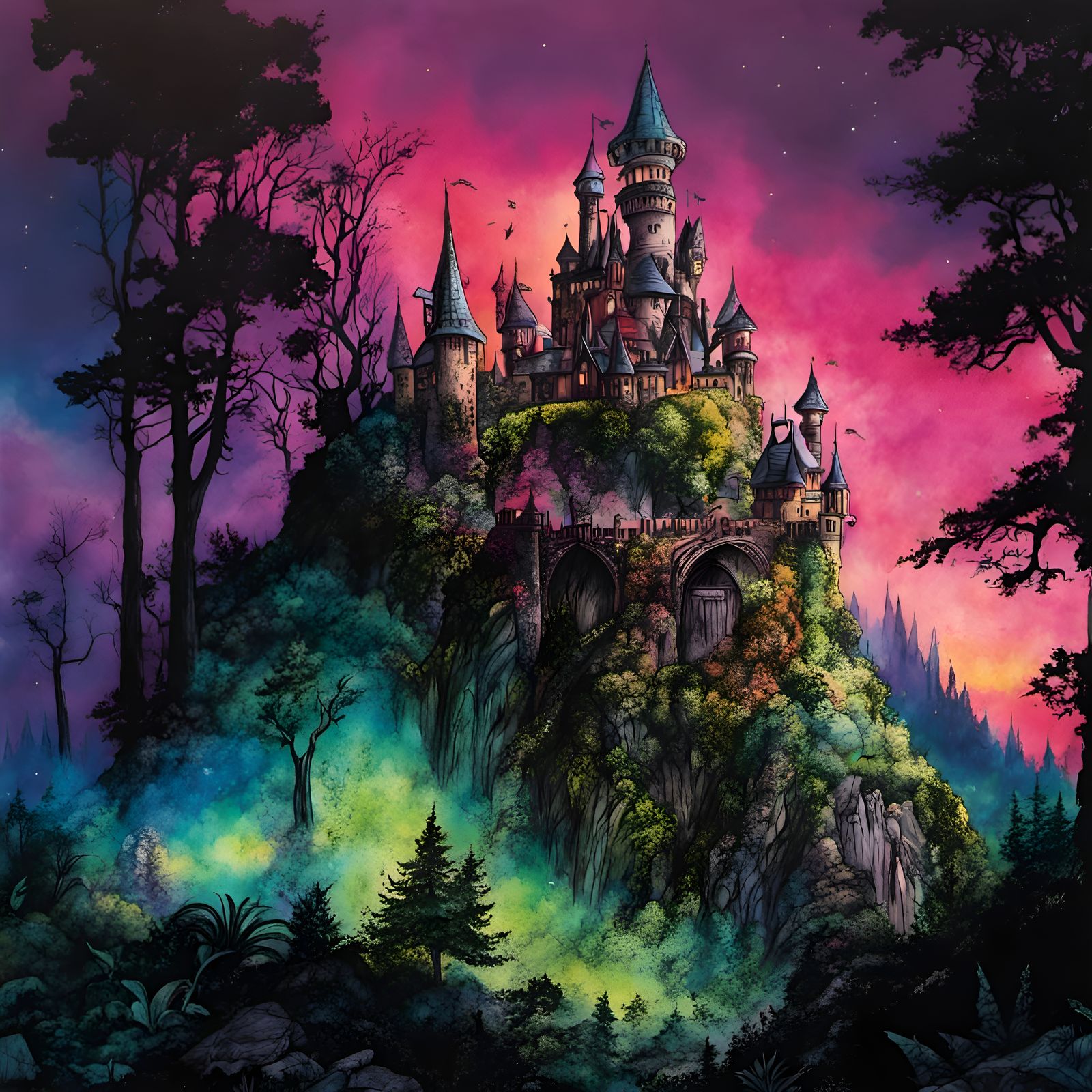This image is an animated cartoon drawing of a grand mythical castle set high upon a mountain top, surrounded by cliffs. The castle is built in multiple stories that stretch down the mountain, becoming more clustered and larger towards the top. Several towers are present, with one particularly large tower in the middle, each adorned with purplish-blue, triangular roofs. The night sky forms a mystical backdrop with hues of pink, purple, and blue, and small star-like dots scattered throughout.

At the base of the mountain, a light green and blue, almost misty fog covers the ground and some of the trees, creating an ethereal atmosphere. Tall pine trees, appearing as black silhouettes in the dim lighting, frame the castle on both the far left and right sides of the image. Some of these trees even reach over the height of the castle. The overall color scheme includes light pinks, blues, and greens, enhancing the fantastical and mysterious ambiance of the scene.